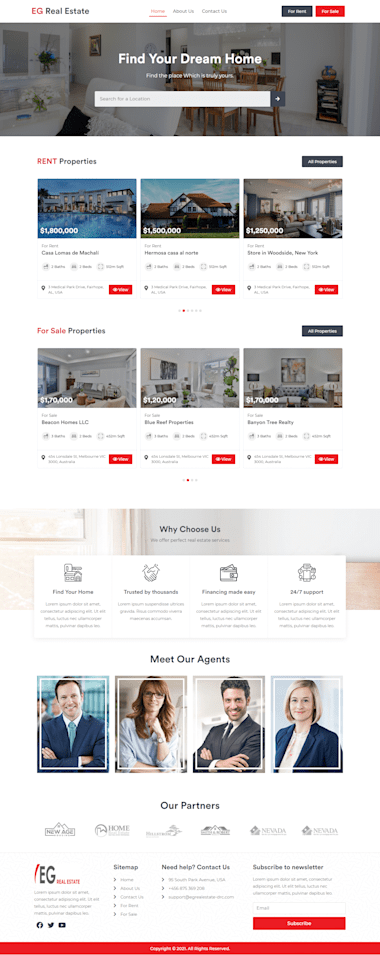The image is an advertisement by Real Estate, titled "Find Your Dream Home." Dominated by a blue title text adjacent to an orange logo, the central feature includes a shaded gray section featuring a search bar prompting users to "Find Your Dream Home" by entering their location. Below, the advertisement showcases rental properties, with the word "Rent" highlighted in orange and "Properties" in blue. This section displays six varied images of rental properties, ranging from the very high-end to more affordable options.

The midsection of the image, subtly colored in light orange, light gray, and white, provides reasons for choosing this real estate company. This section is interactive, allowing users to click through the various reasons. 

Further down, the "Meet Our Agents" section stands out with vibrant imagery of the company's representatives. Featured agents include a distinguished man in a gray suit paired with a teal tie, a woman with reddish hair and glasses, a gentleman in another gray suit with hands folded, and a woman in a gray suit with shorter blonde hair. This group is labeled "Our Partners."

To finalize, an orange "Learn More" button is positioned at the bottom right, inviting further engagement.